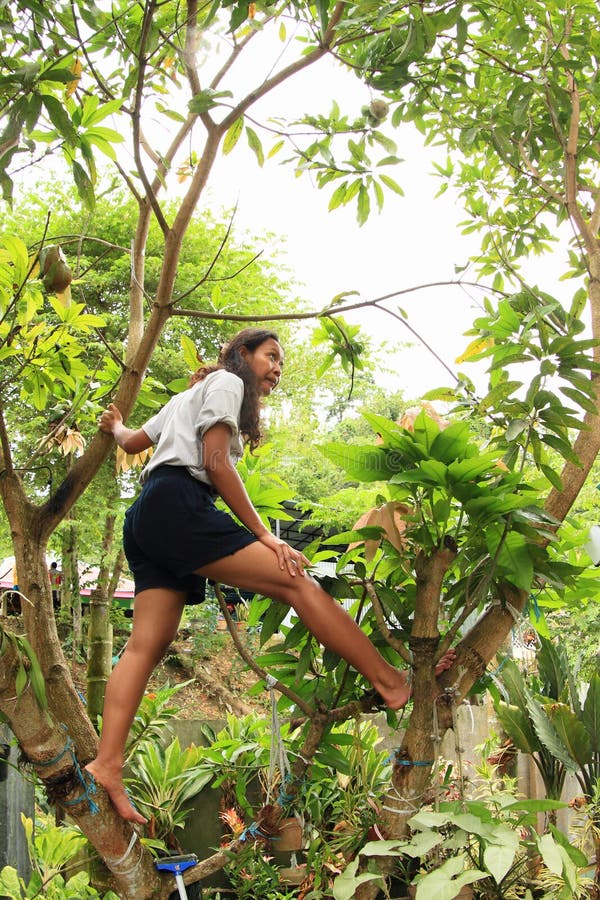In this image, a person with light brown skin and long brown hair is depicted walking barefoot amongst tree branches. They are dressed in a gray t-shirt and black shorts. Their heel is rooted into a spot where one tree branch bifurcates slightly, showing a small area with blue coloring. A nearby branch to the right features a light blue strap wrapped around it. The person might be examining the trees to assess their health, as they seem intent on their surroundings. Above, a gray sky casts a soft light over the scene, which is characterized by the rich brown of the tree branches and the vibrant green of the leaves. On the ground below the person, lies a gray metal stick with a blue tip, possibly used as a tool for their inspection.